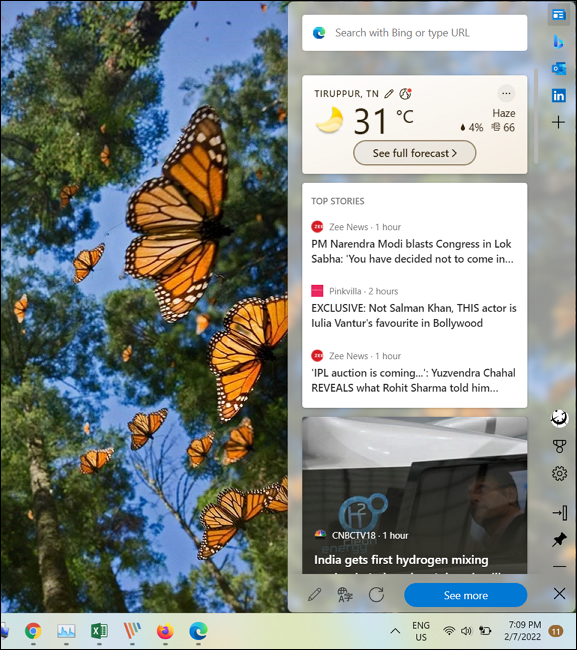A screenshot from a mobile device displaying a colorful scene of monarch butterflies flying amidst tall trees. The viewer’s perspective is from the ground looking up, capturing butterflies at various distances, from nearby to far away. The blue sky provides a vivid backdrop, highlighting the contrasting black and orange of the butterflies, along with the green of the towering trees. On the right side, a light gray overlay partially shades the image. At the top of the screen, a search bar and URL space are featured, followed by a white box indicating the location "Tiruppur, Tennessee," current weather conditions at 31 degrees Celsius with haze, a 4% chance of rain, and unclear symbol representations. Below are the top news stories: Z News reports PM Narendra Modi’s criticism of Congress in the Lok Sabha one hour ago, an exclusive from Pinkville about an actor being Lulia Mantur's favorite Bollywood star two hours ago, and another update from Z News about the upcoming IPL auction.